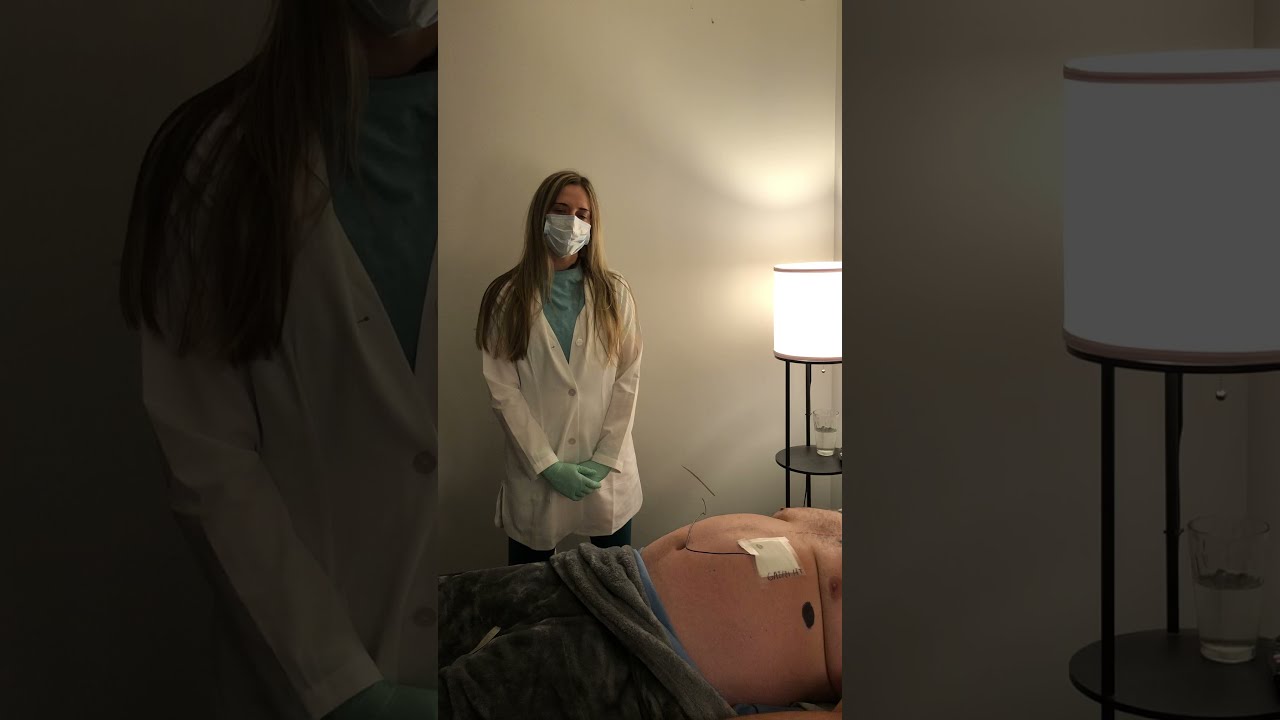The image depicts a medical professional, likely a nurse, standing slightly off-center to the left. She is wearing a white lab coat over a blue shirt, green latex gloves, and a surgical mask. Her long blonde hair is visible behind the mask. The setting appears to be a comfortable, indoor room, potentially designed for medical treatments like acupuncture or post-operative care, rather than a traditional hospital environment. To her right stands a round, glowing white lamp with a black base, which also has a glass of water placed nearby. In front of the nurse, partially visible, is a morbidly obese man lying down, covered with a gray fleece blanket around his midsection. His stomach displays a white gauze patch taped in place, with a wire or tube protruding from his belly button area. There is also a visible scar on his chest, suggesting he might have undergone recent heart surgery. The room features a mix of colors such as off-white, white, yellow, brown, light blue, green, and pink, enhancing its calming ambiance.